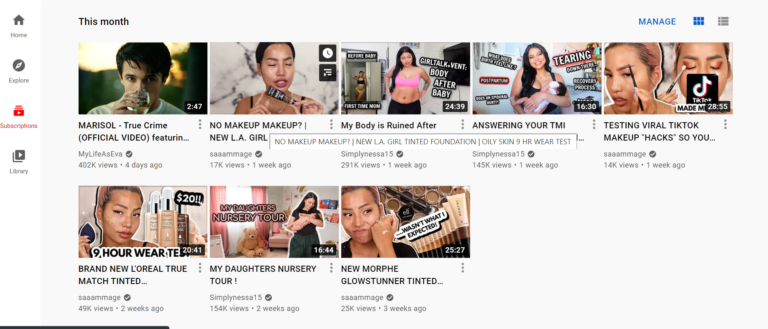**Screenshot of YouTube Subscription Page**

This detailed screenshot captures a YouTube subscription page, showcasing various features and options for personalizing user experience. On the left sidebar, navigation options include Home, Explore, Subscriptions, and Library, with the Subscriptions tab highlighted in red.

The subscription feed reveals recent videos from different channels:

1. "My Life as Eva" presents a video titled "Marisol True Crime Official Video Featuring Someone," adding a thrilling touch to the subscription list for the month.

2. "Simply Nessa 15" is featured multiple times:
   - "No Makeup Makeup: New LA Girl Tinted Foundation Only Skin 9-Hour Wear Test"
   - "Answering Your TMI Questions"
   - "Testing Viral TikTok Makeup Hacks So You Don't Have To: Brand New L'Oreal True Match Tinted" 
   - "My Daughter's Nursery Tours"

3. "Say Saa a Mmage" also makes an appearance with:
   - "My Body is Ruined After Baby"

Finally, users have the option to manage their subscriptions and personalize their viewing preferences, enhancing their overall experience on YouTube.

This detailed caption provides a comprehensive overview of the screenshot, highlighting the variety of content and functionalities available to users.